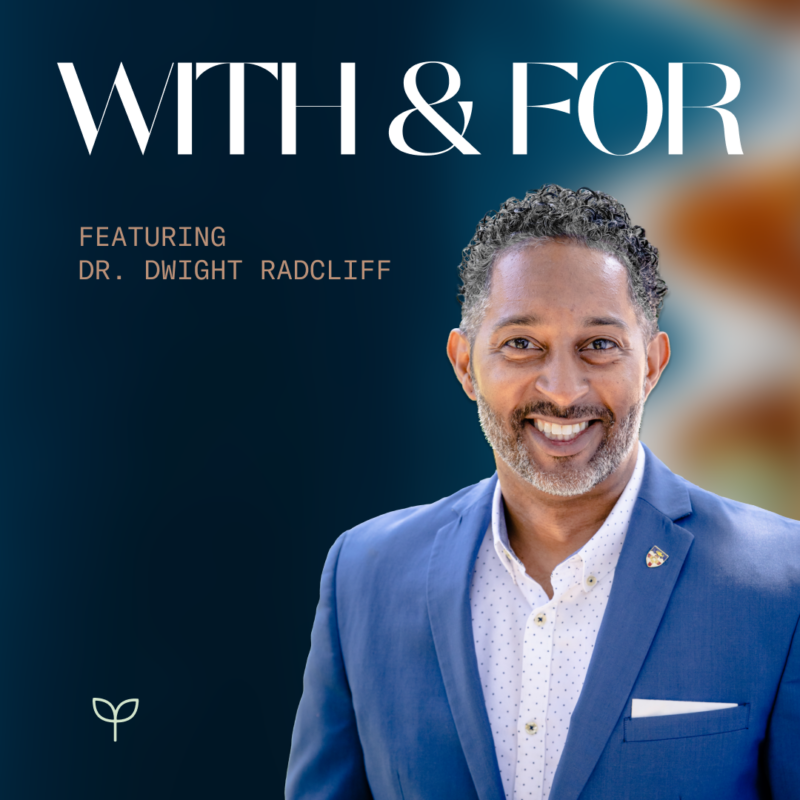This flyer advertises an event titled "WITH AND FOR" in large white text at the top. Below the title, in smaller, salmon-colored all caps, it announces, “FEATURING DR. DWIGHT RADCLIFFE.” The background is primarily dark blue with wavy orange details along the right side. The main focus is on Dr. Dwight Radcliffe, a middle-aged, dark-skinned man with curly black hair graying at the roots, and a small, light mustache and beard. He is smiling and is dressed in a blue jacket with a white button-down shirt. A pin decorates his lapel, and a logo of two stylized leaves is placed at the bottom left of the flyer. The overall design suggests a seminar or speaker event featuring Dr. Radcliffe.